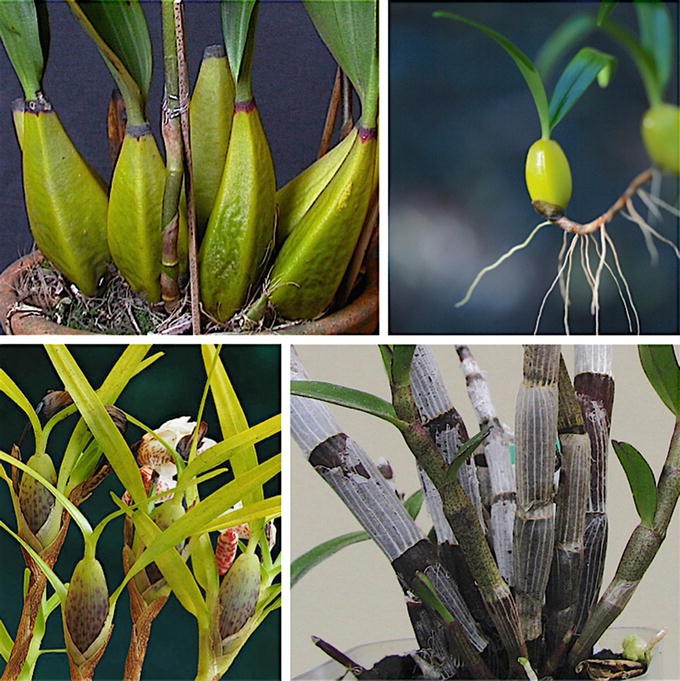In this composite image, there are four photographs of various plant stages and elements arranged in a 2x2 grid. The images on the upper left and lower right are slightly larger than the other two. 

1. **Upper Left**: This photograph depicts the base of a plant with a cluster of lime-green, tuber-like structures emerging from soil. These structures are topped with dark green leaves. The pot's rim is just visible, suggesting these plants are still in the growing phase.

2. **Upper Right**: This image features a thin, brownish root-like branch adorned with a lime-green bulb and two green leaves, suggesting it might be a mature fruit. The background is dark, accentuating the brightness of the plant elements.

3. **Lower Left**: This picture shows another view of the green, leaf-topped structures, potentially depicting the same or similar plants as in the upper left. The leaves are lean and light green, and there are brownish bulbs visible, adding texture to the frame.

4. **Lower Right**: Here, numerous gray and dark brown stems, resembling bamboo with a grayish-white skin, rise together. Only a few leaves are visible, giving it a stark and structured appearance.

Together, these images provide a detailed view of different growth stages and parts of these plants, from tubers and roots to stems and leaves.